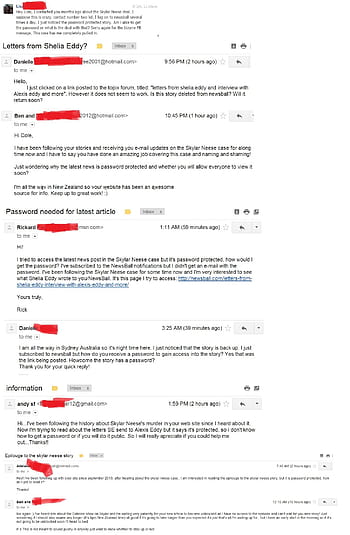This image is a blurred screen capture of a text-based conversation within a social media platform or online forum. Despite significant enlargement, the text remains challenging to decipher. The content is formatted into numerous paragraphs, each separated by a line and marked by user icons on the left, indicating different participants in the discussion. The conversation appears to revolve around letters from Sheila Eddy, with all user information on the right redacted using a thick red marker.

Several distinct usernames, such as Danielle, Ben, Richard, and Rick, are participating in the chat. The large, easily readable titles stand out amidst the unclear text. Towards the bottom of the image, there is a section labeled "Password Needed for Latest Article," accompanied by posts that include timestamps and related information. Another section titled "Information" is present further down. Every name on the left side of the screen is displayed in black, with adjacent redactions obscuring specific details. The redacted content continues consistently throughout the entire page.